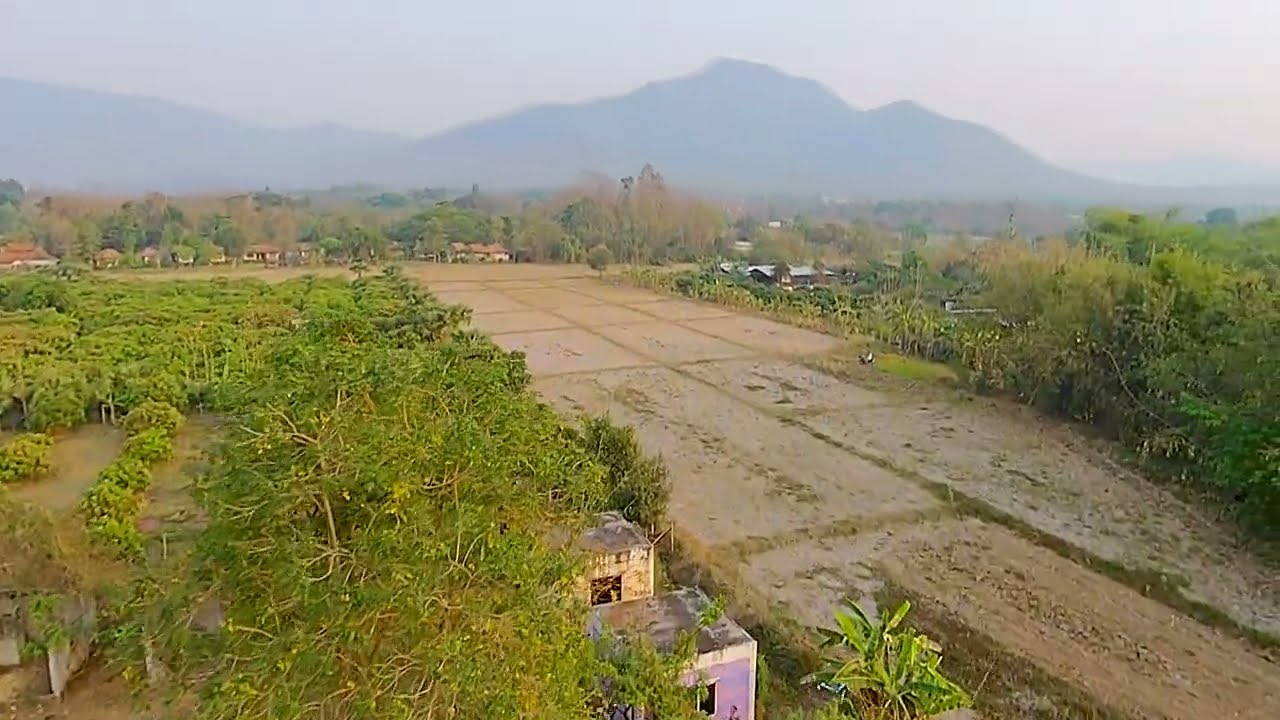This aerial photograph captures a scenic, expansive view of a rural landscape. In the foreground, two blocky pink or rusty buildings with open windows are prominently visible. The viewer's gaze is directed downward, revealing a swath of greenery primarily consisting of dense forests and patches of bushes. These green and light yellow trees are present on both sides of a distinct path, possibly a tiled or dirt road, which bisects the scene horizontally. The path, bordered by rectangular segments of grass, extends toward the horizon where several small houses with orange roofs are nestled.

Further in the background lies a forest showcasing a blend of green and orange foliage, signaling the changing seasons. The terrain appears segmented, possibly from past farming activities or land preparation. Rising majestically beyond the forest is a series of hazy, blue-gray mountains under a dreary, overcast sky. The detailed, layered composition of this photograph effectively merges elements of agriculture, residential life, and natural landscapes, inviting viewers to speculate on its serene yet industrious ambiance.